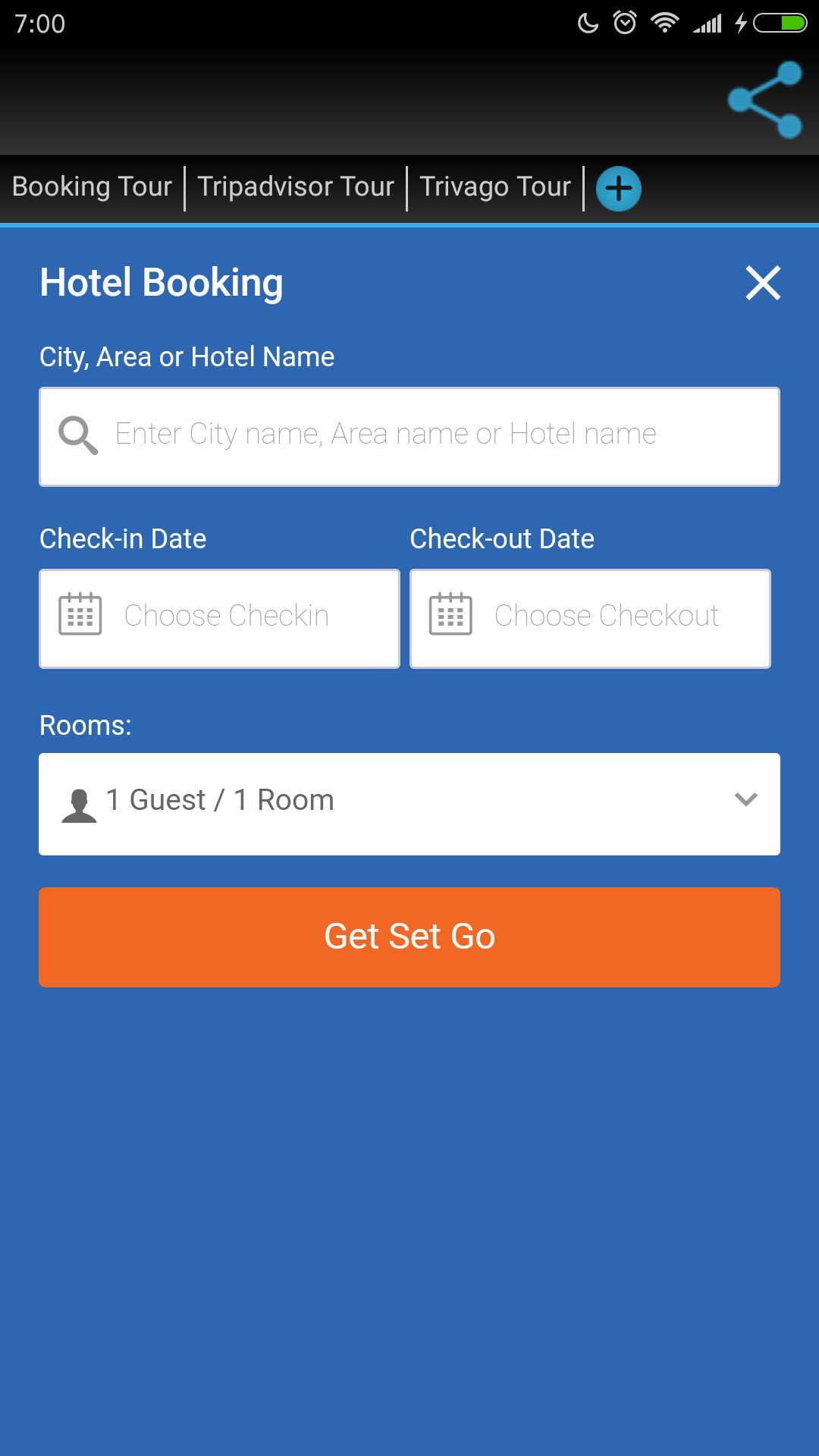This image is a screenshot of a mobile device's screen displaying a hotel booking application interface.

At the top, there is a black bar that transitions to a lighter gray gradient. In the top left corner, the time is displayed as "7:00," in gray lettering. To the right of the time, there are several status icons: a moon icon indicating silent mode, a ringer icon, a Wi-Fi icon, a signal strength indicator, a battery charging icon, and a battery status bar showing half charge with a green and black color split.

Below this bar is a blue header with several elements: the LINE logo (three connected dots) likely for sharing, and a series of tabs for different tour options labeled "Booking Tour," "Trip Advisor Tour," and "Trivago Tour." To the far right is a blue circle with a black plus sign, probably for adding new elements or actions.

The main portion of the screen is dominated by a blue box titled "Hotel Booking." To the right of this title is a white "X" button, presumably for closing the booking interface. Below the title, there is a search box with the placeholder text "City, area, or hotel name."

Under the search box, there are two fields for selecting dates: "Check-in Date" and "Check-out Date," each with a calendar icon for easy date selection. Further down is a section titled "Rooms," featuring a drop-down selector currently set to "1 Guest, 1 Room."

At the bottom of the screen, there is a brightly colored orange bar with the text "GET SET GO" in white letters, indicating the button to initiate the search or booking process.